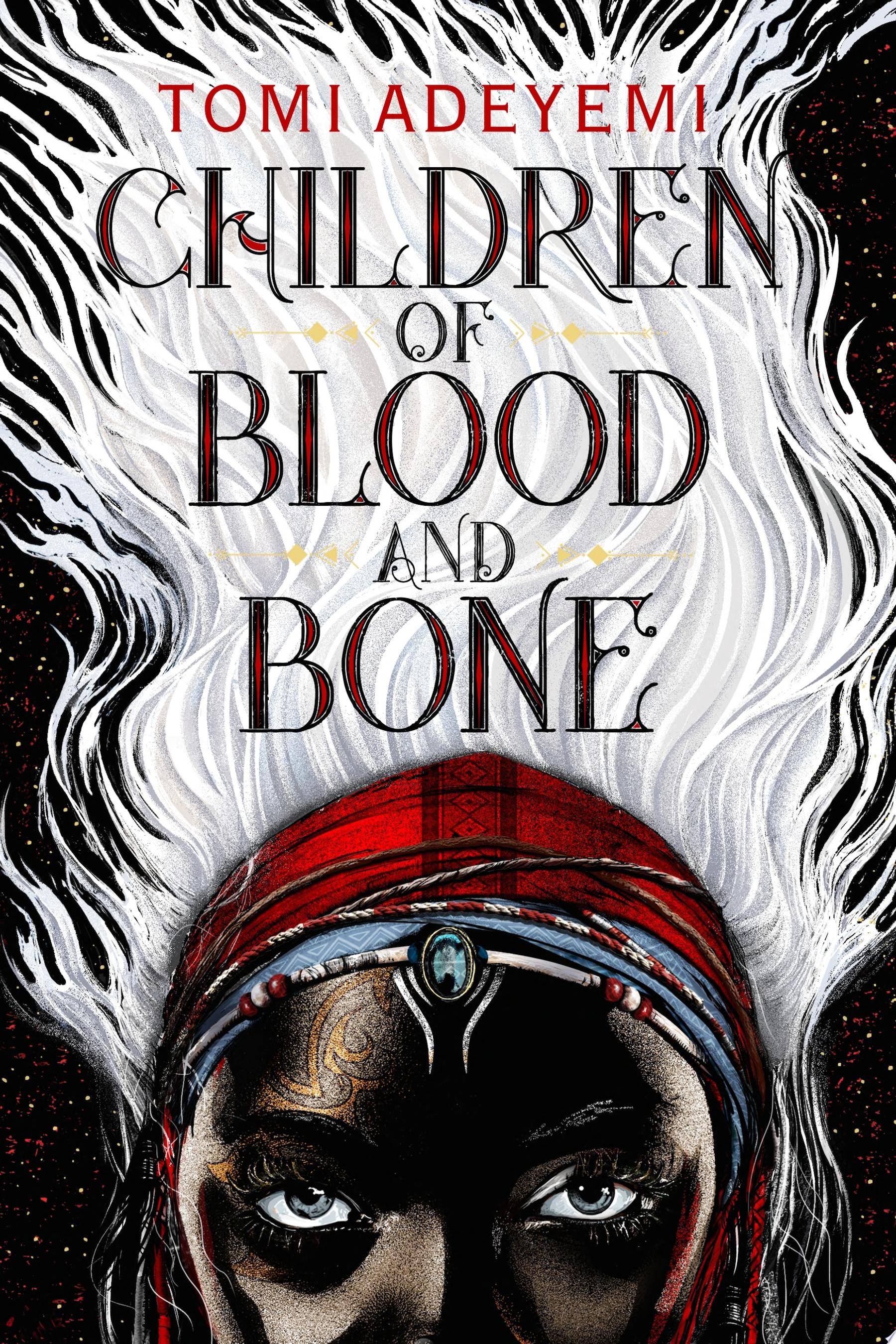The image is a book cover for "Children of Blood and Bone" by Tomi Adeyemi. The title is prominently displayed in an old, biblical style font, with dark red filling framed by a gray or black outline, positioned centrally on the cover. The background is entirely black, accented with small red and white speckles, resembling stars. Dominating the lower part of the cover is the face of a figure, only visible from the nose upwards. The individual's skin is an intense black hue, adorned with gold detailing or tattoos across the left eye and forehead. Their eyes are piercing gray-blue. Adorning their head is an intricate headdress comprised of a red patterned headband, a blue piece underneath, and abundant beads featuring a central turquoise gem. Flowing upwards from the head and occupying a significant portion of the cover is a mass of long, white, airy hair, giving a dynamic, almost ethereal appearance. Behind the figure, there appears to be stylized white smoke or mist, enhancing the mystical aura of the cover design.